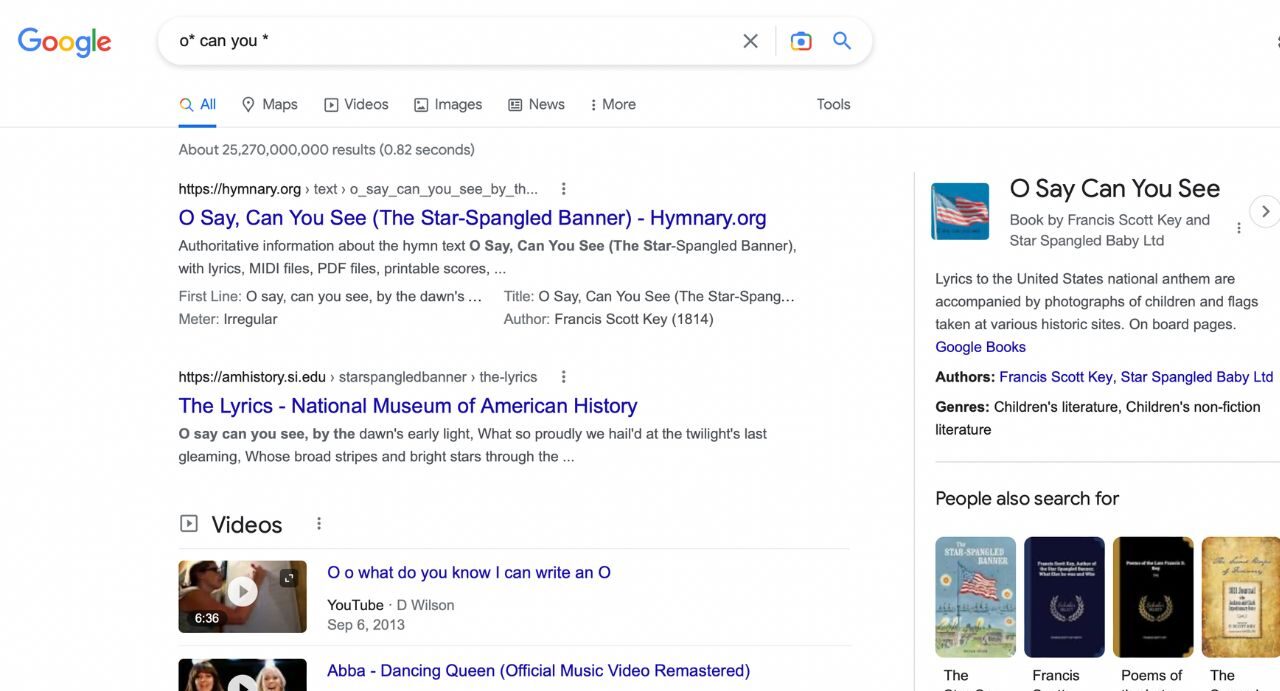The image captures a Google search results page. Prominently displayed in the top left corner is the Google logo, adorned in its signature blue, red, orange, and green hues. Central to the page is the search text box containing the query, which reads "oh can you." Below this, a series of search results are listed, with the titles highlighted in blue text. 

The first result is titled "Oh Say Can You See (The Star-Spangled Banner)" from hymnary.org. The second result, also in blue text, is from the National Museum of American History and is titled "The Lyrics." 

On the right side of the page, there is an image of an American flag flying against a clear blue sky, accompanied by the words "Oh Say Can You See." Directly below, a black text excerpt explains that the lyrics to the United States National Anthem are paired with photographs of children and various flags taken at historic sites, available on Google Books.

Lastly, in the lower section, there is a "People also searched for" section with four rectangles, each seemingly an image of a book. However, the text is too small and blurred to decipher the titles clearly.